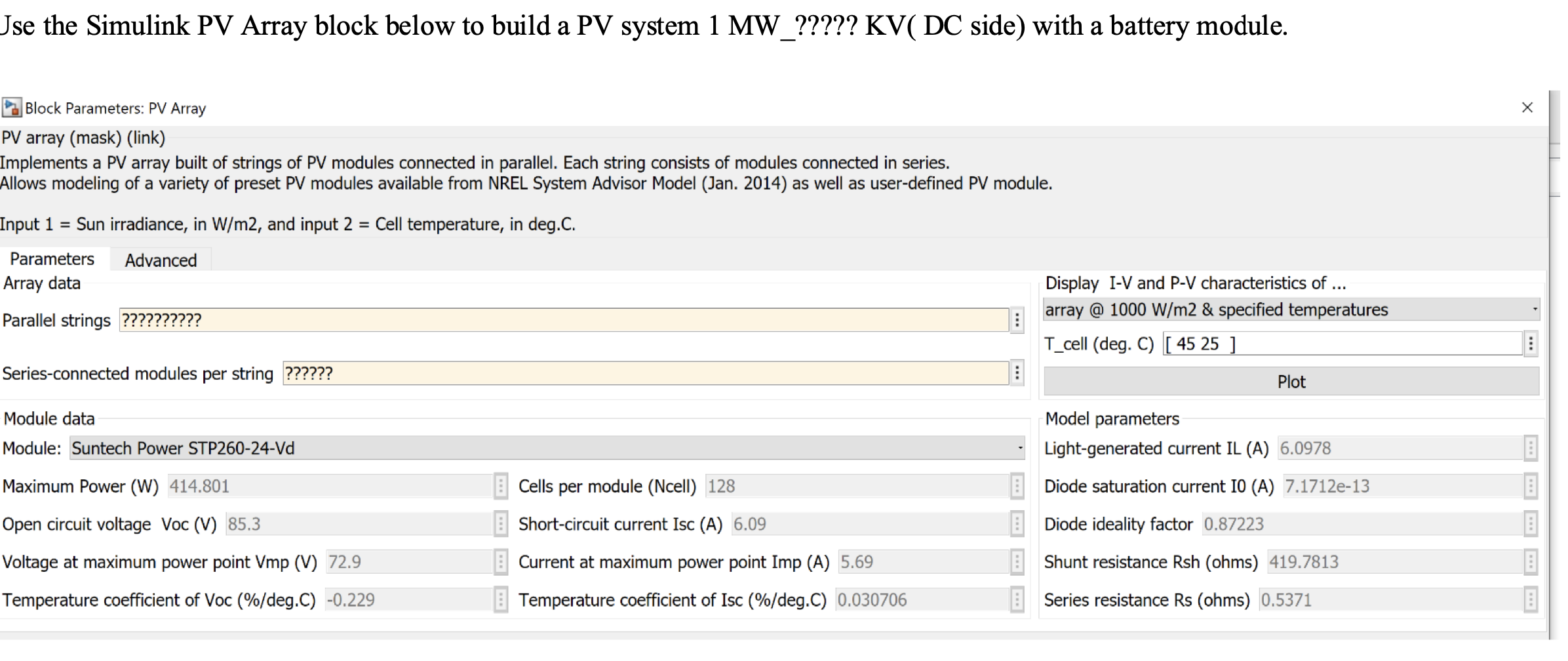**Detailed Caption:**

The image predominantly features a light blue and white background, accented with occasional pink elements within various boxes. At the top of the image, bold black text reads: "JSE, the Simulink PV Array Block Below." It further instructs: "Use the Simulink PV Array Block Below to build a PV system. One MW_????? KV (DC side) with a battery module."

Beneath this heading, a series of boxes in light blue and white with black text are displayed. The first box, a light blue banner, contains the text "PV Array." Inside parentheses, it states "(mask) (link)." The box provides a detailed description: "Implements a PV array built of strings of PV modules connected in parallel. Each string consists of modules connected in series. Allows modeling of a variety of preset PV modules available from NREL System Advisor Model (January 2014), as well as user-defined PV modules."

Following this description, additional black text specifies: "Input 1 = Sun irradiance in W/M², Input 2 = Cell temperature in °C."

Below this explanation, there are two pink boxes meant for entering array data parameters. The first pink box is labeled "Parallel strings" and contains several question marks. The second pink box, labeled "Series connected modules per string," also contains several question marks. Additional boxes are provided below these for further data entry.